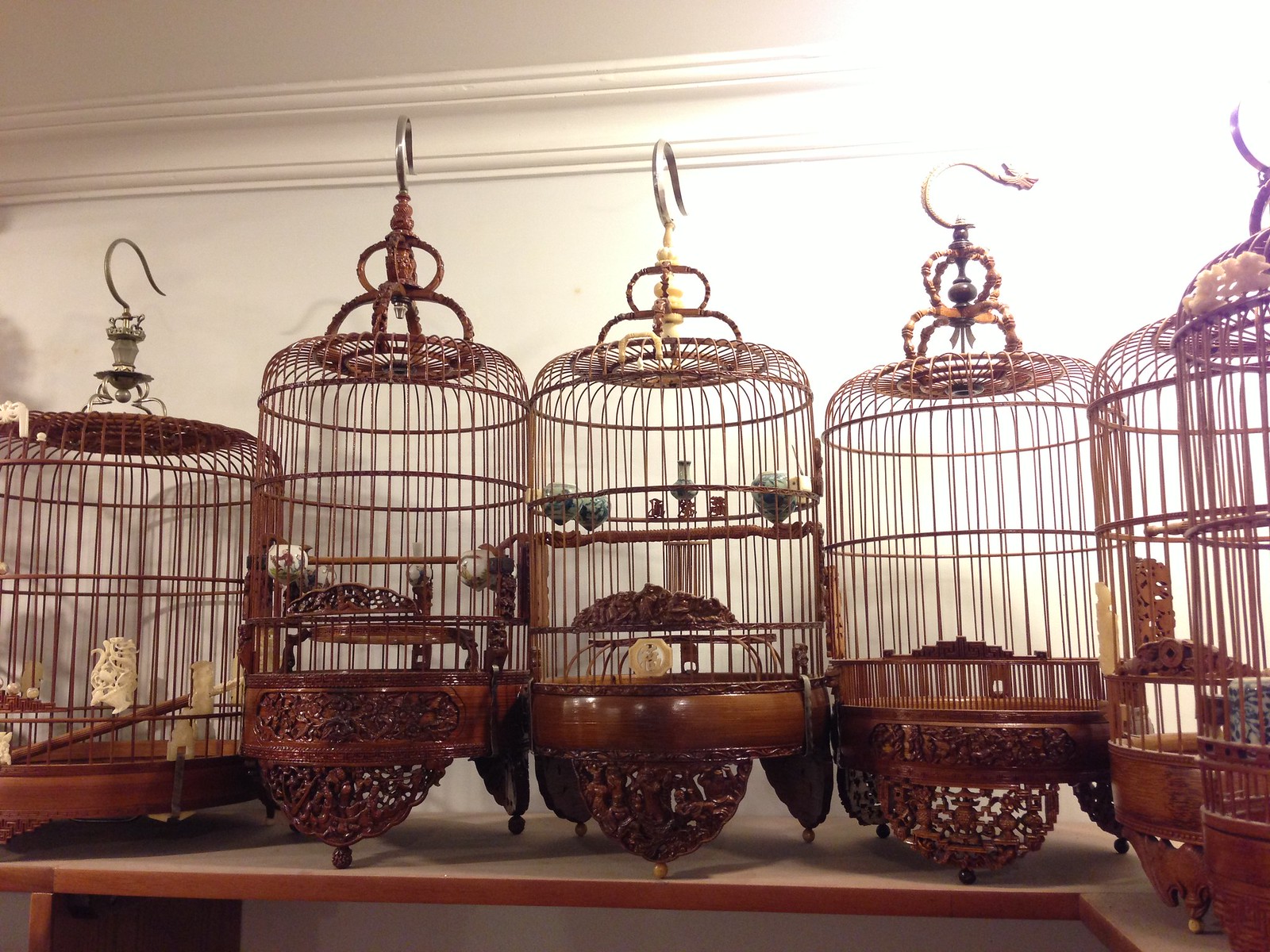This detailed photograph captures six intricately crafted vintage bird cages, prominently displayed on a wooden table with a lightly colored brown trim. A very bright light shines from the upper right-hand corner, illuminating the scene against a backdrop of a white wall, adorned with white crown molding and a white ceiling. The cages, made predominantly of cherry brown wood, stand out for their unique design, where even the traditional wire components are fashioned from wood. 

All six bird cages, with most appearing nearly identical, are exquisitely ornate. The three middle cages are particularly notable for their scrollwork, filigree, and a two-tiered hook design, possibly adorned with beads. The overall aesthetic is completed by elegant frilly designs carved into the wood at the base of each cage, suggesting their vintage and possibly expensive nature. 

Inside the cages, no live birds can be found; instead, there are decorative items such as fake birds and what appears to be an ivory carving, indicating their likely use for display. This carefully staged arrangement, possibly inside a home or a store, underscores the beauty and craftsmanship of these wooden bird cages.